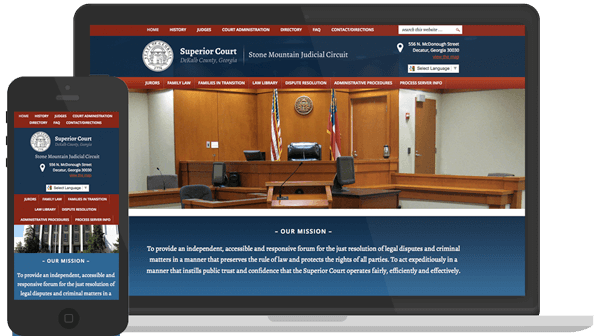A split-screen image compares the mobile and desktop versions of the Superior Court Stone Mountain Judicial Court website. The desktop version, displayed on a laptop, features a structured layout with a red banner at the top, followed by a blue section labeled "Superior Court," additional menu options in another red banner, and an interior photo of the court. Below the image, the mission statement is prominently displayed in white letters on a blue background.

In contrast, the mobile version, viewed on a smartphone, adapts to the smaller screen with a red banner at the top, the same "Superior Court" title, and dropdown menus for navigation. Beneath this, there is an image of the state capitol building, followed by the mission statement. The fonts remain consistent between both versions, maintaining a cohesive look with red and blue color schemes. This image effectively highlights the design differences between the two platforms while showcasing the same informative content.